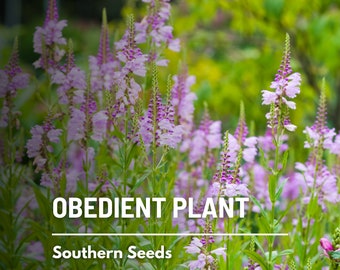The image is an outdoor, rectangular photograph featuring a cluster of obedient plants (Physostegia virginiana), with delicate, lavender-colored flowers blooming along tall, slender green stems. The focal point of the photo showcases these elegant, purple-hued flowers, which resemble small lavender cattails, arranged horizontally and framed by a background of blurred green foliage. The top left corner of the image is darker, creating a gradient effect that fades into the brighter, sunlit area where the flowers are more visible. In bold white capitalized letters, the label "OBEDIENT PLANT" is prominently displayed at the top of the photograph, with a horizontal line beneath it and the phrase "Southern Seeds" written below. This visually detailed presentation suggests it could be part of a web page or an advertisement for gardening products.